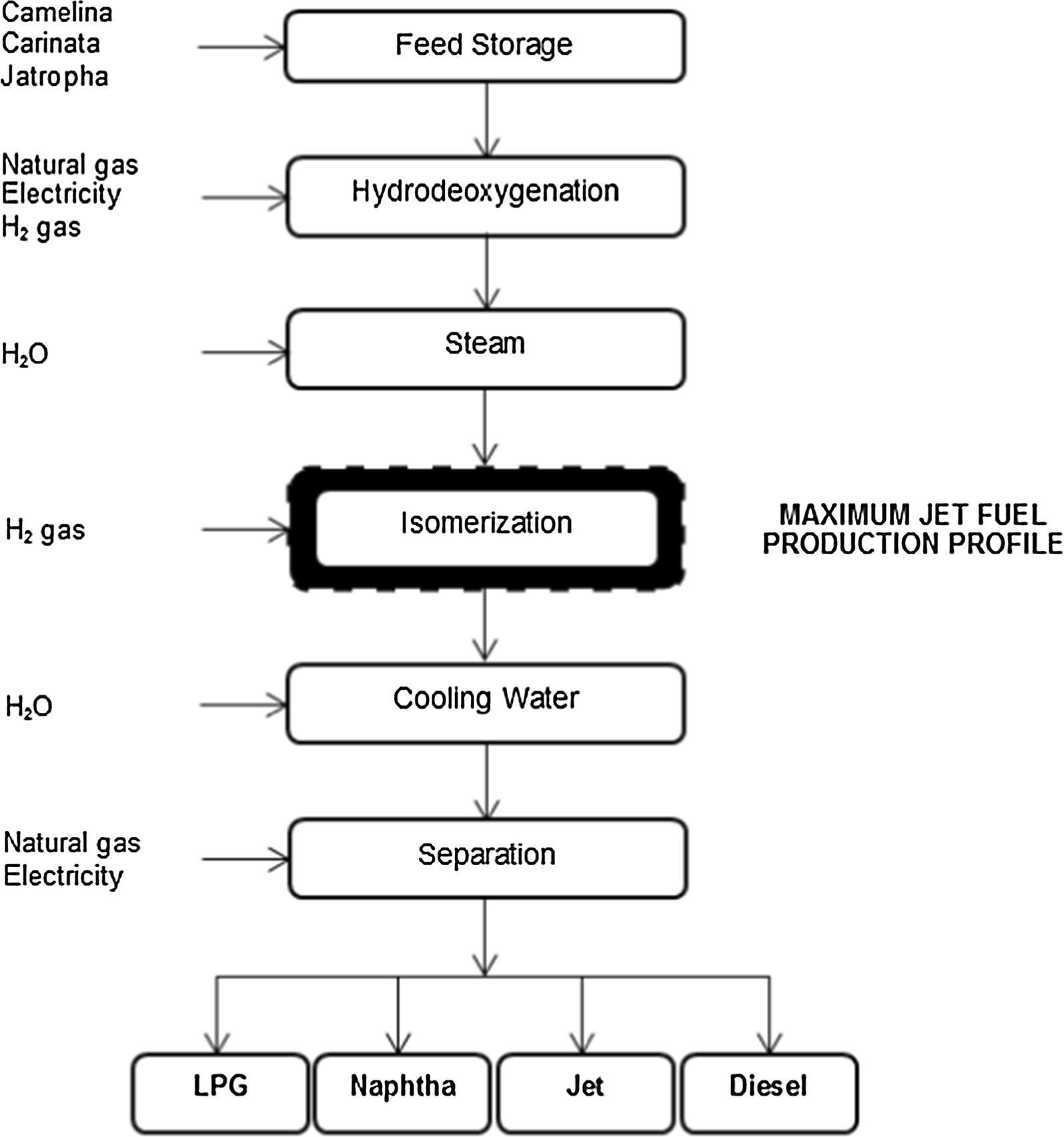The image features a detailed black-and-white diagram illustrating a multi-step process flow for fuel production. The central portion of the diagram is populated with rectangular bars connected vertically by arrows, leading from top to bottom. The sequence starts with "Feed Storage," followed by "Hydro Deoxygenation," "Steam," "Isomerization," "Cooling Water," and "Separation." The final stage broadens into four separate items labeled "LPG," "Naphtha," "Jet," and "Diesel."

Accompanying each stage on the left side are specific inputs needed for the processes:
- "Feed storage" is aligned with "Camelina, Karanata, Jatropha."
- "Hydro Deoxygenation" requires "Natural Gas, Electricity, H2 Gas."
- "Steam" is associated with "H2O."
- "Isomerization" notes "H2 Gas.”
- "Cooling Water" associates with "H2O."
- "Separation" requires "Natural Gas, Electricity."

On the right side of the diagram, adjacent to "Isomerization," is a noteworthy label in all caps: "MAXIMUM JET FUEL PRODUCTION PROFILE." The diagram is entirely devoid of colors, additional borders, or any figures, maintaining a straightforward and technical presentation.